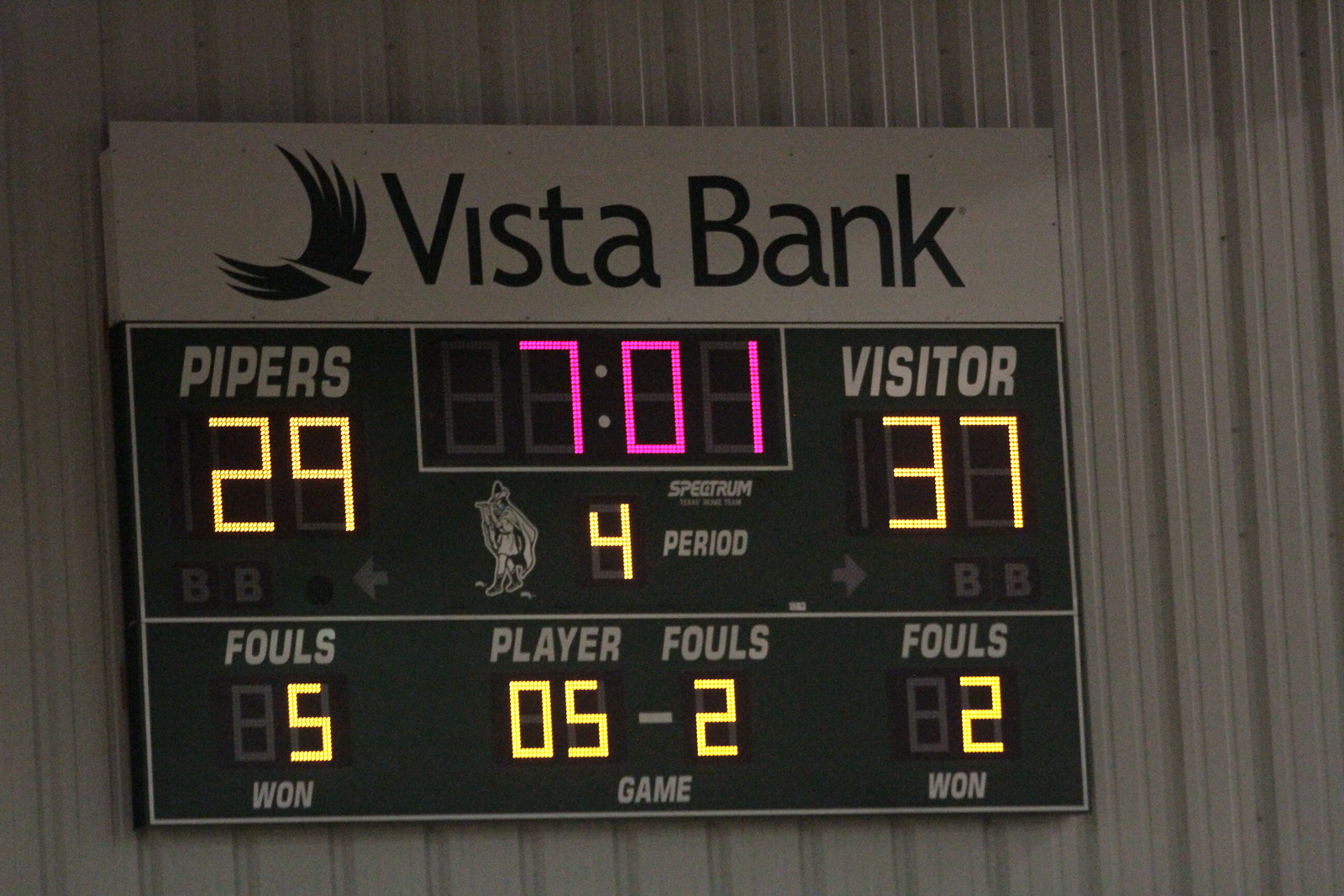The close-up photograph captures an electronic scoreboard, mounted on a sheet metal wall typical of a gymnasium. At the top, it displays "Vista Bank" alongside a stylized bird logo. Below, the scoreboard reveals "Pipers 29" to the left and "Visitor 37" to the right, indicating the current scores for a school sport event. The clock in the center displays seven minutes and one second remaining. The period is marked as "4," and adjacent to this is an image of a Pied Piper playing a pipe. Foul counts are detailed, with "Pipers" having five fouls and "Visitors" having two. Additionally, the "Players and fouls" section indicates "0:5" for Pipers and "2" for Visitors. The scoreboard is prominently displayed, with its vibrant details contrasting against the plain white metal wall, illuminated by adequate lighting, and devoid of any other visible objects in the scene.